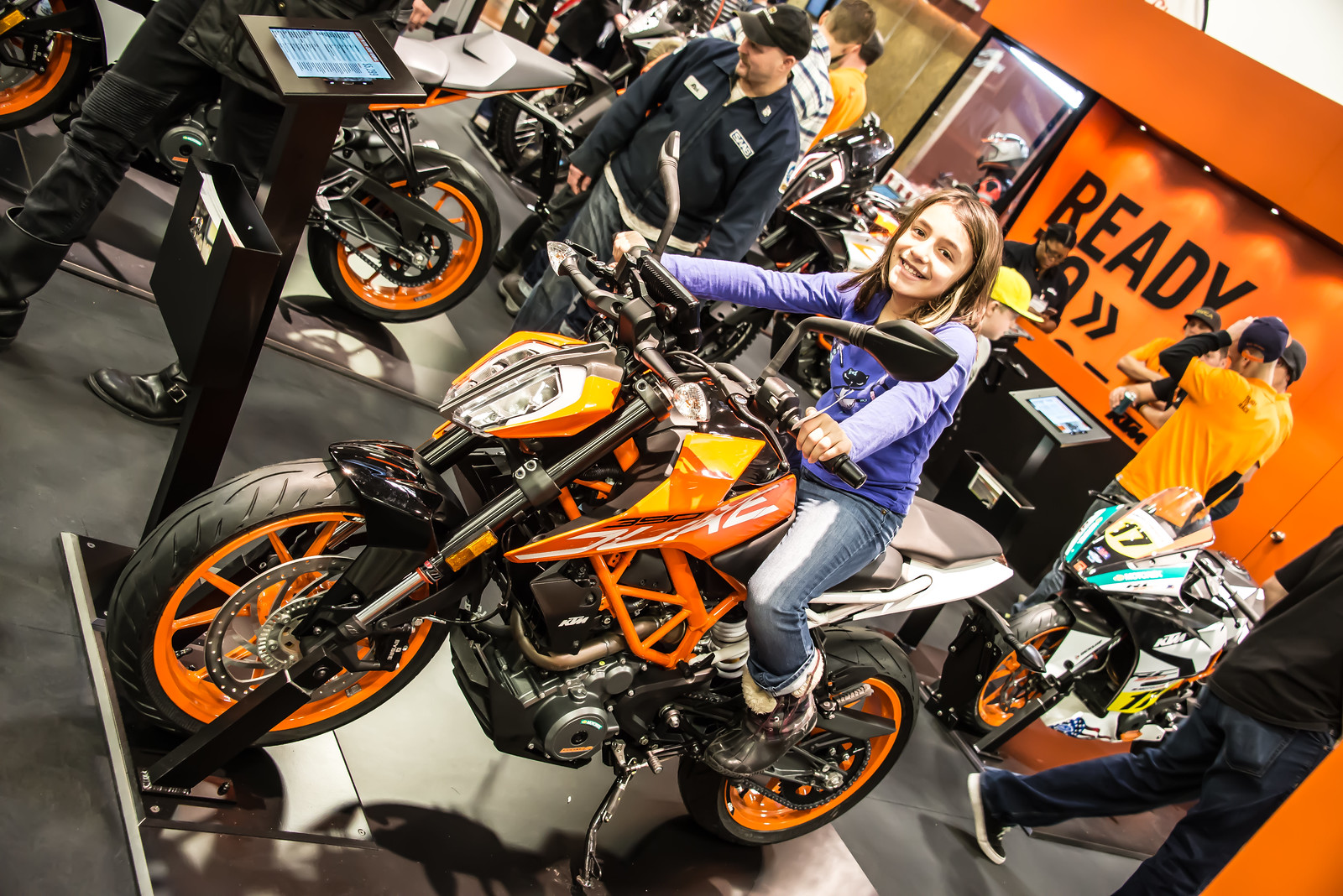In this indoor showroom filled with various motorcycles, a young preteen girl with shoulder-length, straight brown hair is straddling an orange and black motorbike that is displayed on a platform. Dressed in a long-sleeve lilac blue shirt, jeans, and black fur-trimmed boots, she poses confidently with her hands gripping the handlebars, giving the impression that she's ready to ride. The showroom has an orange wall in the background with the word "READY" prominently displayed in black letters. Around her, several other motorcycles are visible on similar platforms, hinting at a store that specializes in these vehicles. The bustling scene includes a man wearing a baseball cap, another gentleman in a yellow t-shirt seemingly embracing someone in a purple knit cap, and about seven or eight other people scattered around. Among them, a man stands just behind the girl, his attention directed towards another motorcycle, seemingly unrelated to her. The image captures a lively moment, with the young girl's excitement and the vibrant showroom setting beautifully framed in a dynamic angle.